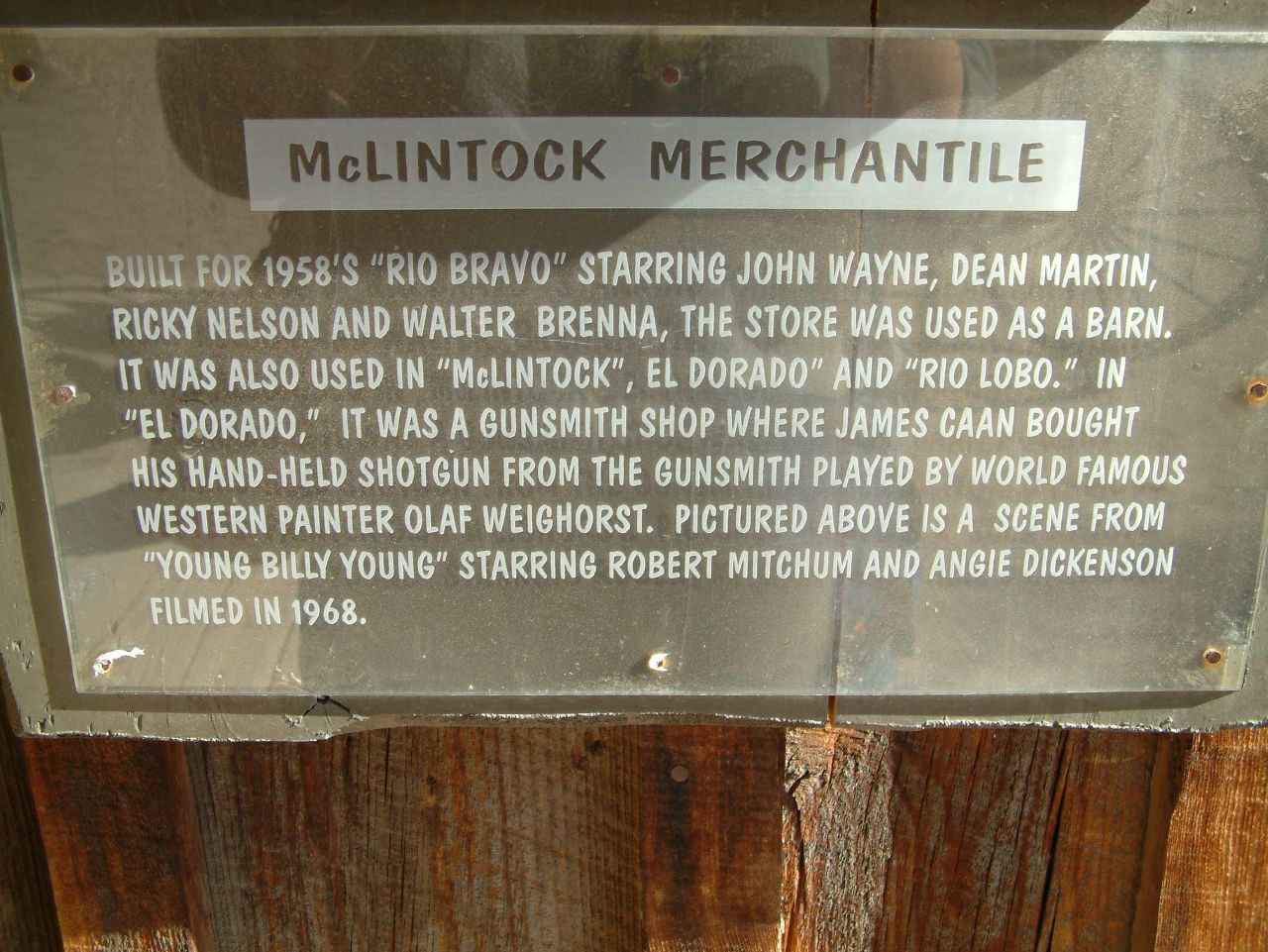This image features an informational sign firmly attached to a rugged wall composed of dark brown logs. The sign, made of clear plastic with white and gray printing, is rectangular and wide. At the top, it reads "McClintock Mercantile." The detailed paragraph below states that the building was constructed for the 1958 film "Rio Bravo," which starred John Wayne, Dean Martin, Ricky Nelson, and Walter Brennan, where it served as a barn. The building was subsequently utilized in several other films: "McClintock," "El Dorado," and "Rio Lobo." Notably, in "El Dorado," it functioned as a gunsmith shop where James Caan's character purchased a handheld shotgun from a gunsmith portrayed by the renowned Western painter Olaf Weighorst. The sign also mentions that a scene from the 1968 movie "Young Billy Young," featuring Robert Mitchum and Angie Dickinson, is pictured above.